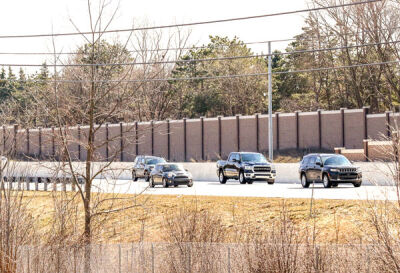This color photograph captures a bright, shiny outdoor scene, likely by the side of a highway or interstate on the side of a hill. The road is flanked by a light brown, high sound wall or fence. In the foreground, there's a dirt road with a chain-link fence and brown vegetation. The area boasts numerous trees, most of which have bare branches, indicating it may be winter or a cold season, though some trees in the background still retain green foliage.

Four black vehicles are driving along the road. Leading the convoy is a black SUV, followed by a black pickup truck, a Fiat Mini Cooper, and another smaller black SUV or sedan. The entire scene is framed by telephone lines strung overhead and a utility pole with a guardrail next to the road. The sky shows some cloud coverage, and the overall image has a slight yellow tint, possibly from evening light. There are no visible people, animals, buildings, or text in the photograph.